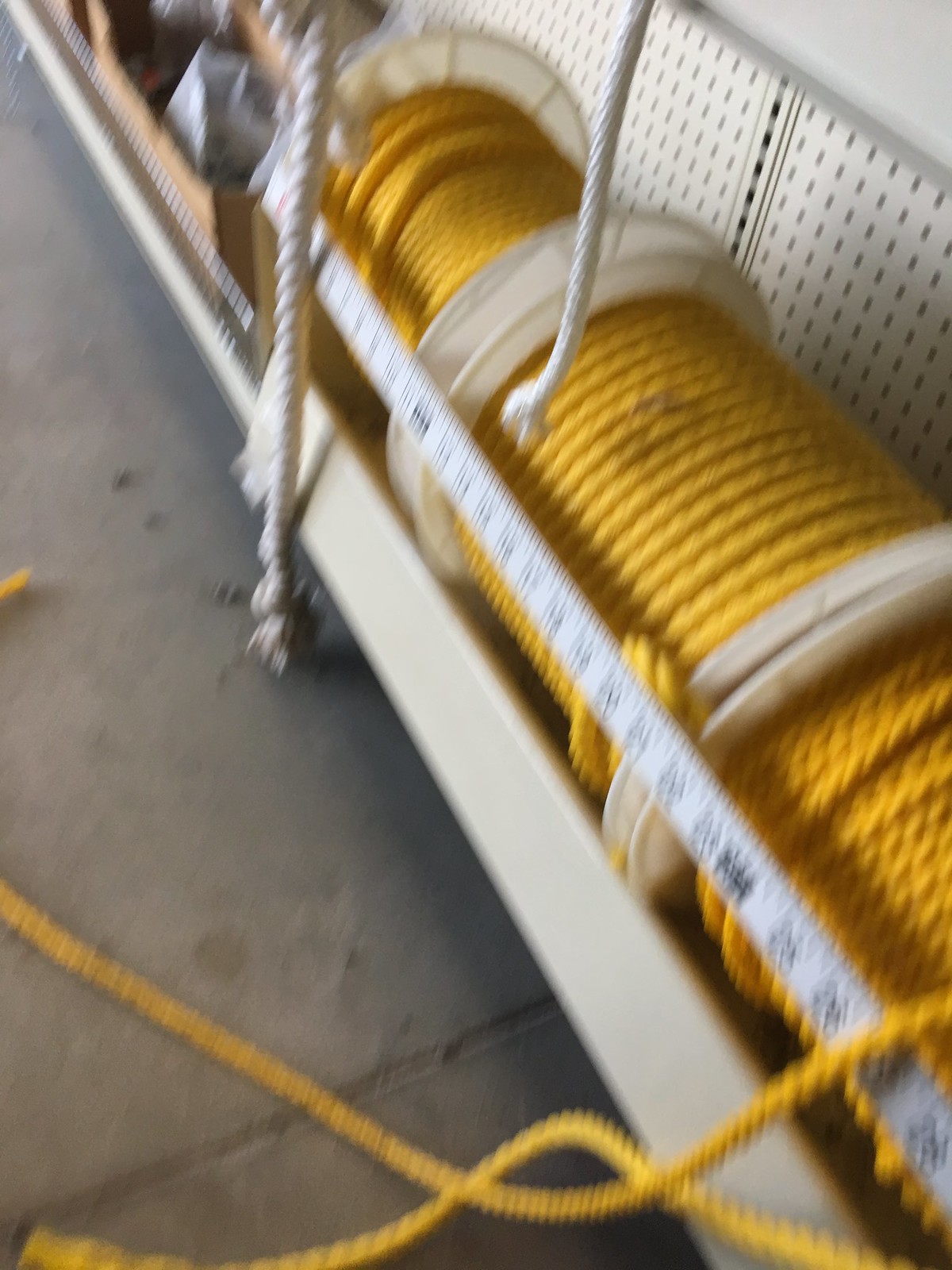On a sturdy concrete base, a shelf stands against a backdrop of industrial metal, displaying three large, thick spools of vibrant yellow rope. The spools are arranged diagonally, stretching from the bottom right corner to the upper left of the image. Above them, an upper shelf holds white rope, with two strands cascading down. Loose pieces of yellow rope unfurl from the front spool, trailing onto the adjacent gray sidewalk. A measuring tape or line is positioned in front of the spools, adding a sense of scale and precision to the vibrant, industrial scene.